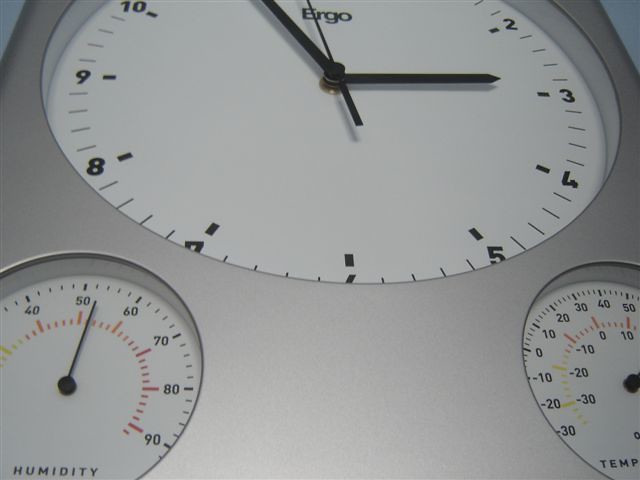In the image, there is a prominently displayed clock with two additional gauges. The scene is somewhat unconventional, as none of the instruments are fully in view, but their primary details are discernible. The main clock, encased in a silver housing, features Arabic numerals and indicates a time of approximately 2:55 or 3:55. Adjacent to this clock is a humidity sensor, its single dial showing a humidity level slightly above 50%. Although the temperature gauge is partially cropped out of the frame, it is evident that the temperature reading exceeds 60. The overall composition creates a somewhat enigmatic atmosphere, as the exact mounting or placement of these devices is unclear.